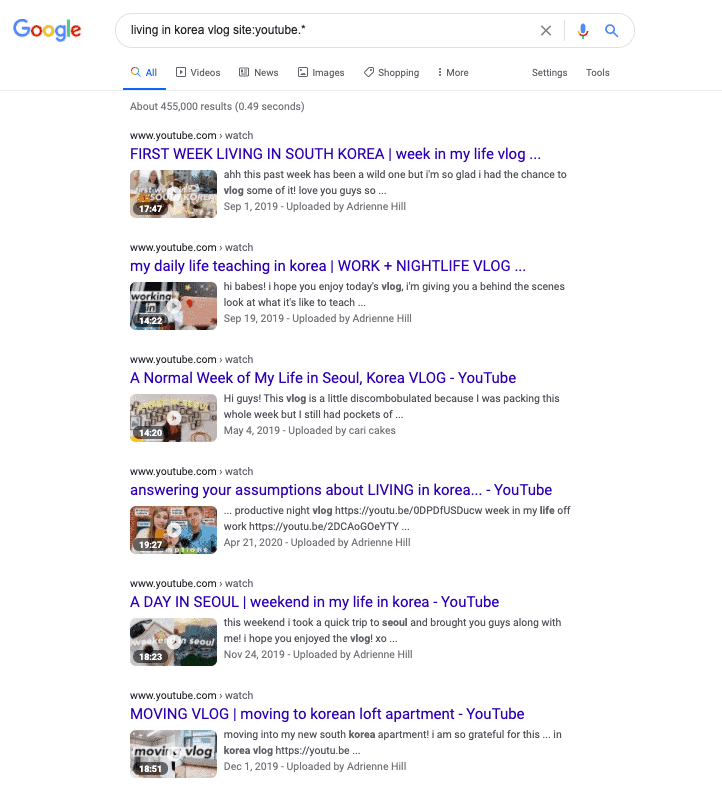Screenshot of a Google Search Results Page for "Living in Korea Vlogs"

In the screenshot, a Google search results page is displayed from the desktop version. The search query "living in Korea vlogs site:youtube.com" has been entered into the search bar at the top of the page. The Google logo is visible at the top left corner against a white background. The search yielded approximately 455,000 results.

Prominent among the results are thumbnails of YouTube videos recommended based on the search query. Here are the top two entries:

1. **First week living in South Korea | Week in my life vlog**
   - **Description**: "This past week has been a wild one, but I'm so glad I had a chance to vlog some of it. Love you guys."
   - ** Duration**: 17 minutes and 47 seconds

2. **My daily life teaching in Korea | Work plus nightlife vlog**
   - **Description**: "Hi babes, I hope you enjoy today's vlog. I'm giving you a behind-the-scenes look at what it's like to teach..."
   - **Duration**: 14 minutes and 22 seconds

Additionally, there are four more video results displayed on the first page, all of which appear to be updated predominantly by an individual named Adrienne Hill.